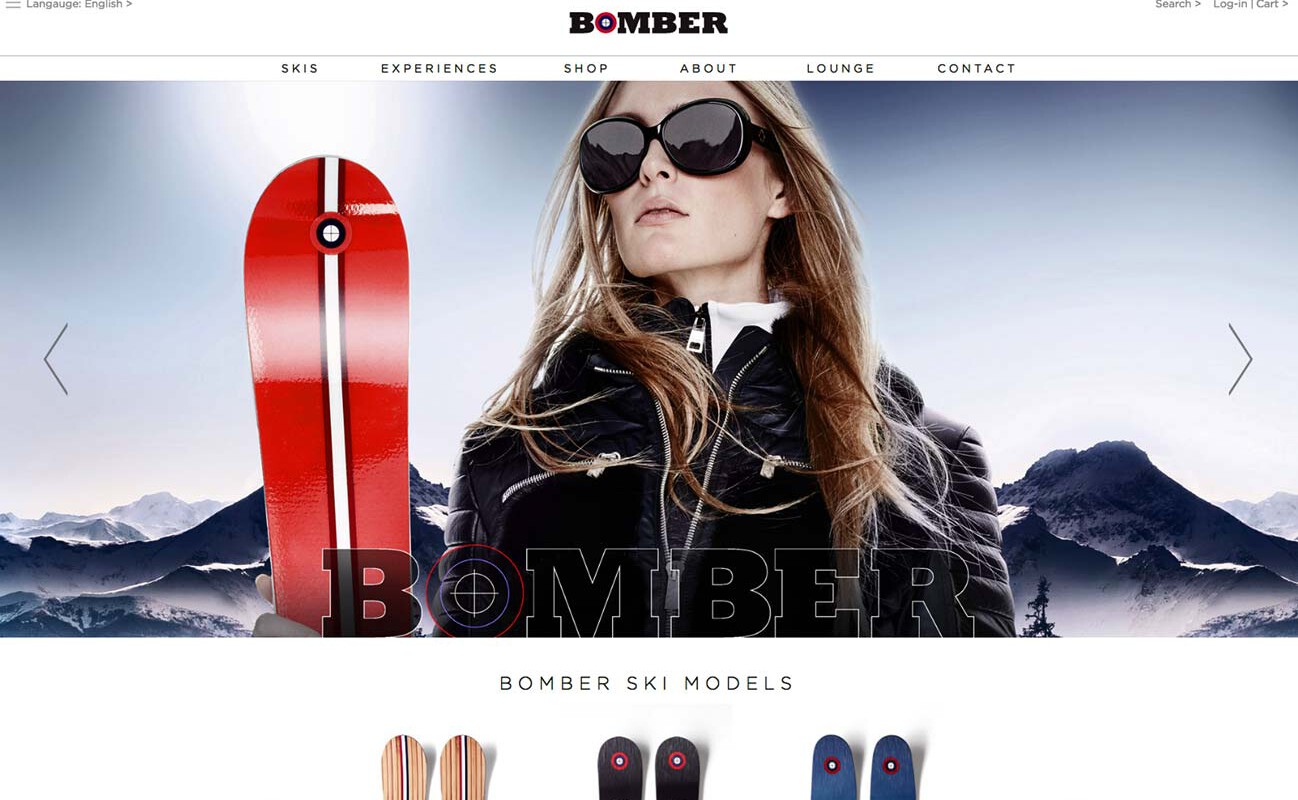The image appears to be a screenshot from a product webpage for Bomber Ski Models. At the top, there is a white banner featuring navigation options such as "skis," "experiences," "shop," "about," and more. The Bomber logo, written in black, features a distinctive red bullseye for the letter "O." The main focal point is a blonde woman with large, dark sunglasses, wearing an unzipped black winter jacket. She is standing in front of snow-covered mountains and holding a red pair of skis. At the bottom of the image, there is text that reads "Bomber Ski Models," accompanied by the tips of three different sets of skis in various colors.